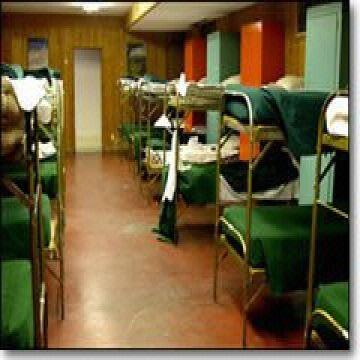The photograph depicts a well-organized barracks room with multiple rows of bunk beds lined against the walls. The floor is a light brown linoleum, showing signs of wear with various gray spots. The bunk beds, which feature rectangular mattresses covered with thick green sheets, are neatly arranged—five visible on the right and three on the left. A mix of personal items adds slight individuality to the otherwise uniform beds. The top bunks appear less orderly, with green blankets hanging down and white sheets more visible.

The room includes alternating green and orange lockers on the right, extending towards the background where a wooden archway frames a white door. A white-and-black handheld vacuum cleaner leans against one of the bunks. The photograph is set against a white background with a thin black border framing it, creating a floating effect enhanced by shadows cast on the bottom and right sides. The overall impression is of a military-style dormitory designed for mass accommodation, characterized by its clean lines and orderly arrangement.